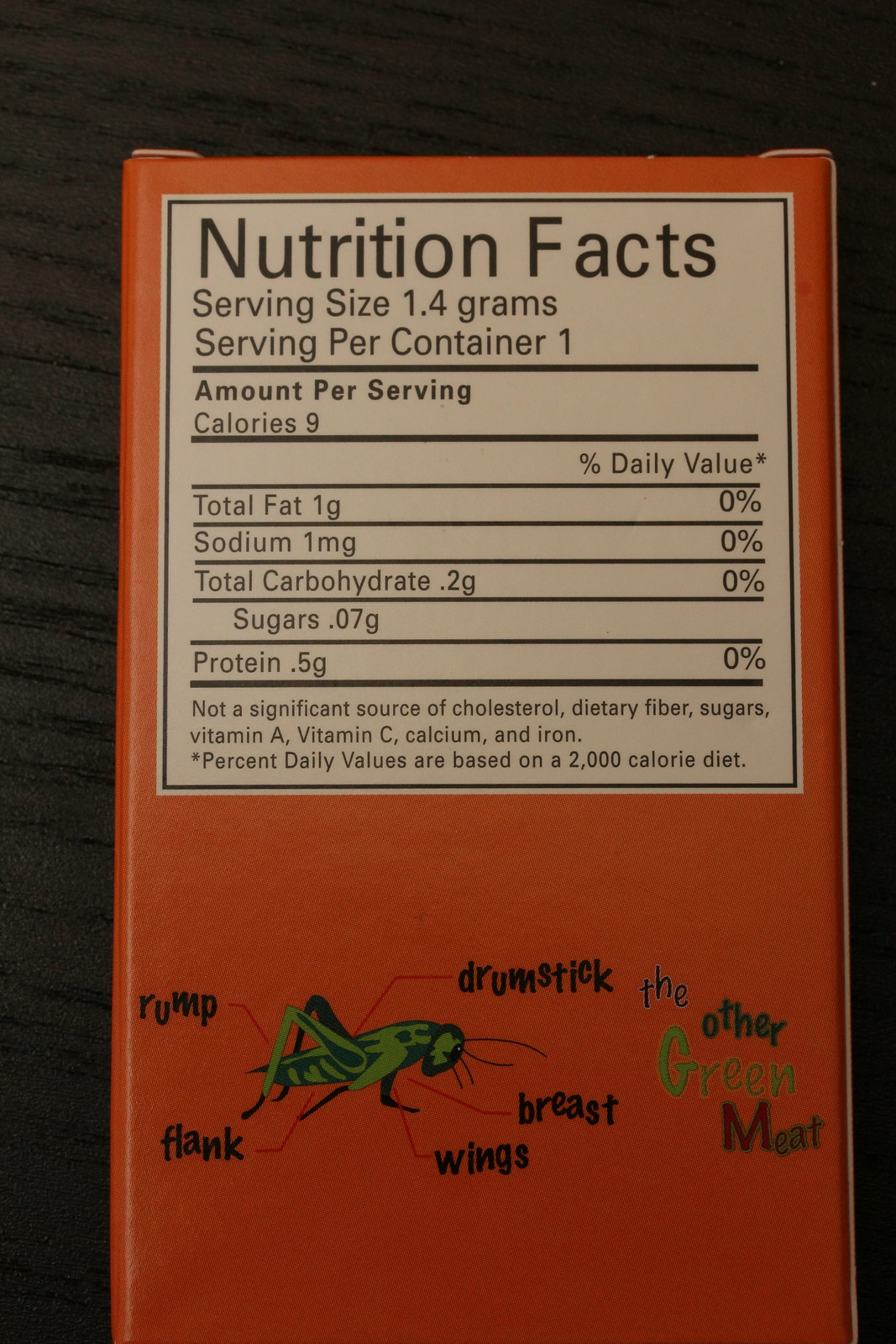The image features a unique and intriguing orange label prominently displaying nutritional facts on a clean, white table. Below this white section, the orange background serves as a canvas for a detailed illustration of a grasshopper. The grasshopper is depicted with various segments of its body labeled with names commonly associated with meat cuts, such as "rump," "flank," "wings," "breast," and "drumstick." The grasshopper appears poised as if it might hop away at any moment. The nutritional information specifies "Serving per container: 1" and "Serving size: 1.4 grams," suggesting that the label is likely from a single-serving packet rather than a tub.